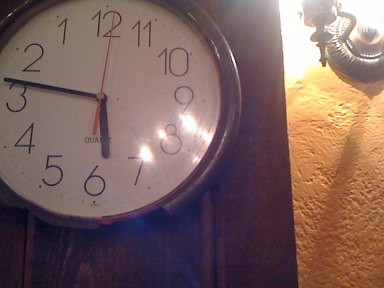This detailed color photograph captures a close-up of a distinctive clock mounted on a dark brown wooden background. Dominating approximately two-thirds to three-quarters of the image, the clock features a dark brown wooden frame, though the bottom of the frame appears to be broken. The clock face is a whitish hue, accented with black hour and minute hands, and a striking red second hand. Notably, the numerals on the clock are arranged counterclockwise, creating an unusual effect where the positions of traditional numbers are reversed (for example, where you typically find 11 is now a 1, and where you expect 10, there is a 2). Adding to the vintage feel of the image, there are small dots of light on the right side of the clock face, contributing to its grainy texture. To the right of the clock, an orange textured carpet extends upwards to the blown-out white upper right corner of the photograph. There, a roundish metallic object, possibly a vacuum or a decorative sconce, partially intrudes into the frame. The juxtaposition of these elements enhances the intriguing character and nostalgic aesthetic of the composition.